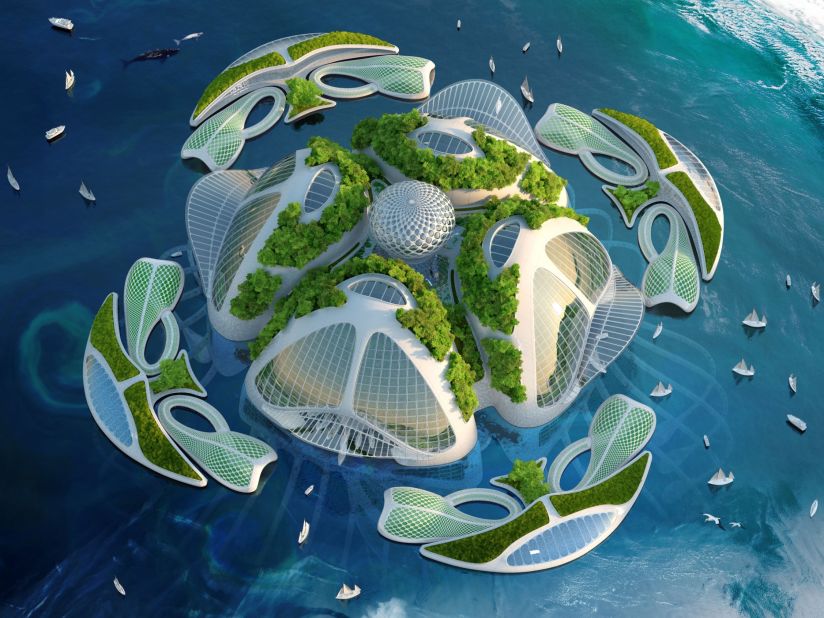This image is an aerial rendering of a futuristic city nestled in the ocean, representing a vision of Aquarius. At the center of the city lies a globe-like structure, surrounded by four ultra-modern buildings adorned with solar panels and abundant greenery. These buildings appear to hover above the water, but their foundations extend deep below the surface. Encircling this central hub are four identical smaller islands, each independent yet mirroring the sustainable design ethos of the main island. The entire scene is dotted with numerous sailboats, which accentuate the expansive scale of the area. In the top left corner of the picture, a large black whale alongside a smaller white whale adds a touch of nature to the futuristic setting, while gentle waves lap in the top right corner, completing this innovative aquatic metropolis.